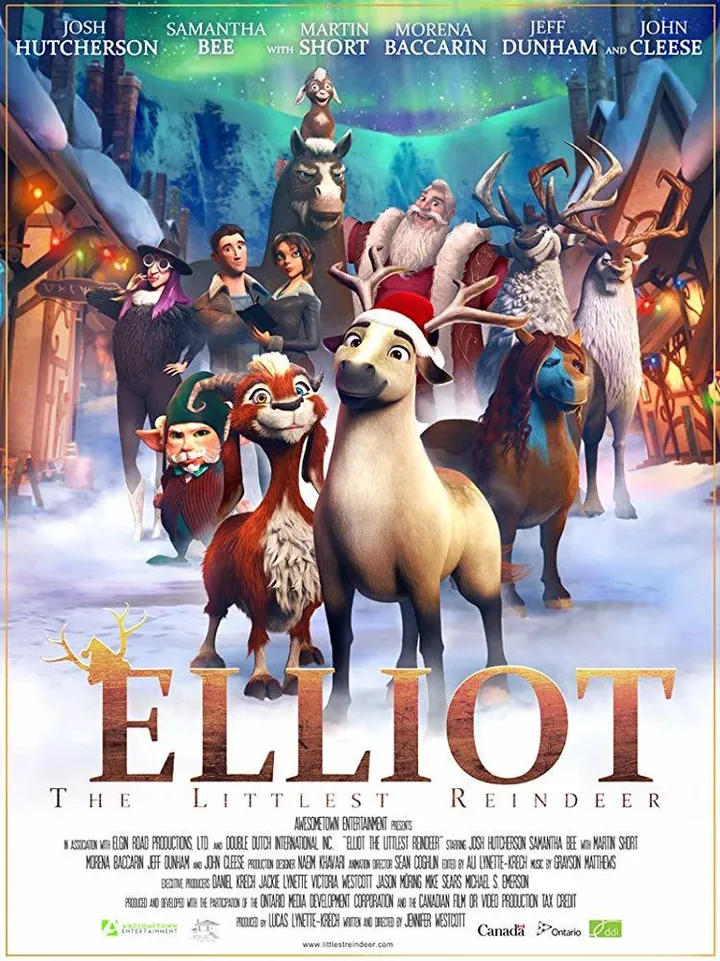The movie poster for "Elliot, The Littlest Reindeer" prominently features cartoon characters and is adorned with vibrant holiday elements, suggesting a North Pole setting. Central to the image is Elliot, a small, tan and brown reindeer with delicate antlers, black eyes, and a black nose. He is accompanied by a small, orange and white-furred mammal with one blue eye and one green eye. Surrounding them is a festive scene with Santa Claus clad in his iconic red suit, flanked by a donkey and reindeer with large antlers. To the sides, colorful houses adorned with Christmas lights add to the holiday ambiance. Several human characters appear in the background, including one dressed like a hippie witch, and a small elf with green eyes and a matching green hat. The top of the poster lists the film's stars: Josh Hutcherson, Samantha Bee, Martin Short, Marina Baccarin, Jeff Dunham, and John Cleese. Below the title, additional production credits are noted, emphasizing the collaborative effort behind the animated holiday film.